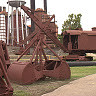The image is a very small, three-quarters of an inch square photograph of an outdoor scene. It features what appears to be various brown items that resemble farming or old machinery equipment, possibly including a catapult-like structure or something that swivels. The items are situated on grass, and the predominant colors in the image are tan, brown, green, and white. There is no text and no people visible in the picture, and the background includes a tree and some indiscernible structures. Notably, one of the items has a circular, upside-down dome shape attached to its top, and there is a walking path visible in the lower right corner. The overall impression is of outdated or abandoned equipment, possibly relics from a past era.